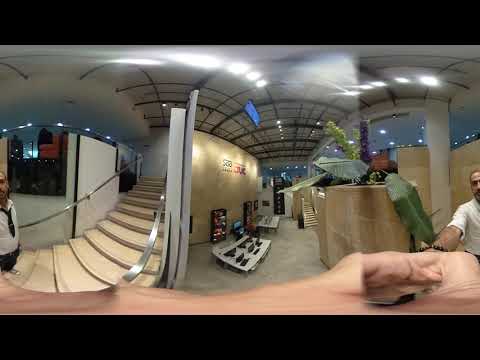The photograph, seemingly taken indoors with a fisheye lens effect, captures a detailed scene in what appears to be an office or possibly a restaurant. Central to the image is a wide-angle view looking back towards the photographer, whose arm is partially visible at the bottom, suggesting the use of a selfie stick. The photographer's arm, wearing a bracelet and a white shirt, intrudes into the shot. 

Just left-of-center, there's a beige stairway with sleek silver handrails, constructed from wood plank flooring, leading up to a second level. Standing at the base of this staircase is a middle-aged man dressed in a white, short-sleeved, unbuttoned shirt exposing a black t-shirt underneath, accompanied by black pants. He has salt-and-pepper hair and is positioned in the bottom right corner of the image.

The space further to the right appears more cluttered and distant, showing tables or shelves against the wall. The ceiling overhead features bright white rectangular lights. The far-right side of the image includes large green leaves, possibly from ferns or banana plants, enhancing the otherwise office-like environment with a touch of greenery. The walls are a muted beige color, and the floor is gray. In addition, there are black objects and vending machines lined up along the beige walls on the left side, further furnishing the setting.